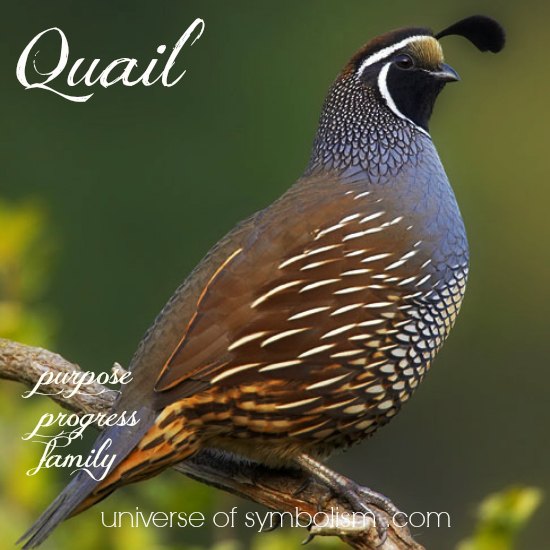This is a detailed photograph of a quail, prominently positioned in the center. The bird is perched on a small brown tree limb against a blurred, dark green background, enhancing the quail's visual prominence. The quail's body predominantly features brown feathers with specks of white near the wings. As you observe the neck and head, the brown feathers gradually turn black. The head is mostly black with a few strips of white. A distinctive black feather extends from the base of its head. Only one of its eyes and its beak are visible.

At the top left of the image, the word "quail" is elegantly scripted in white cursive font. Below this, on the bottom left, are the words "purpose," "progress," and "family," also in white cursive. Finally, at the very bottom center of the image is the website name "universeofsymbolism.com." This card-like image beautifully blends the detailed depiction of the quail with symbolic text elements, reinforcing themes of purpose, progress, and family.